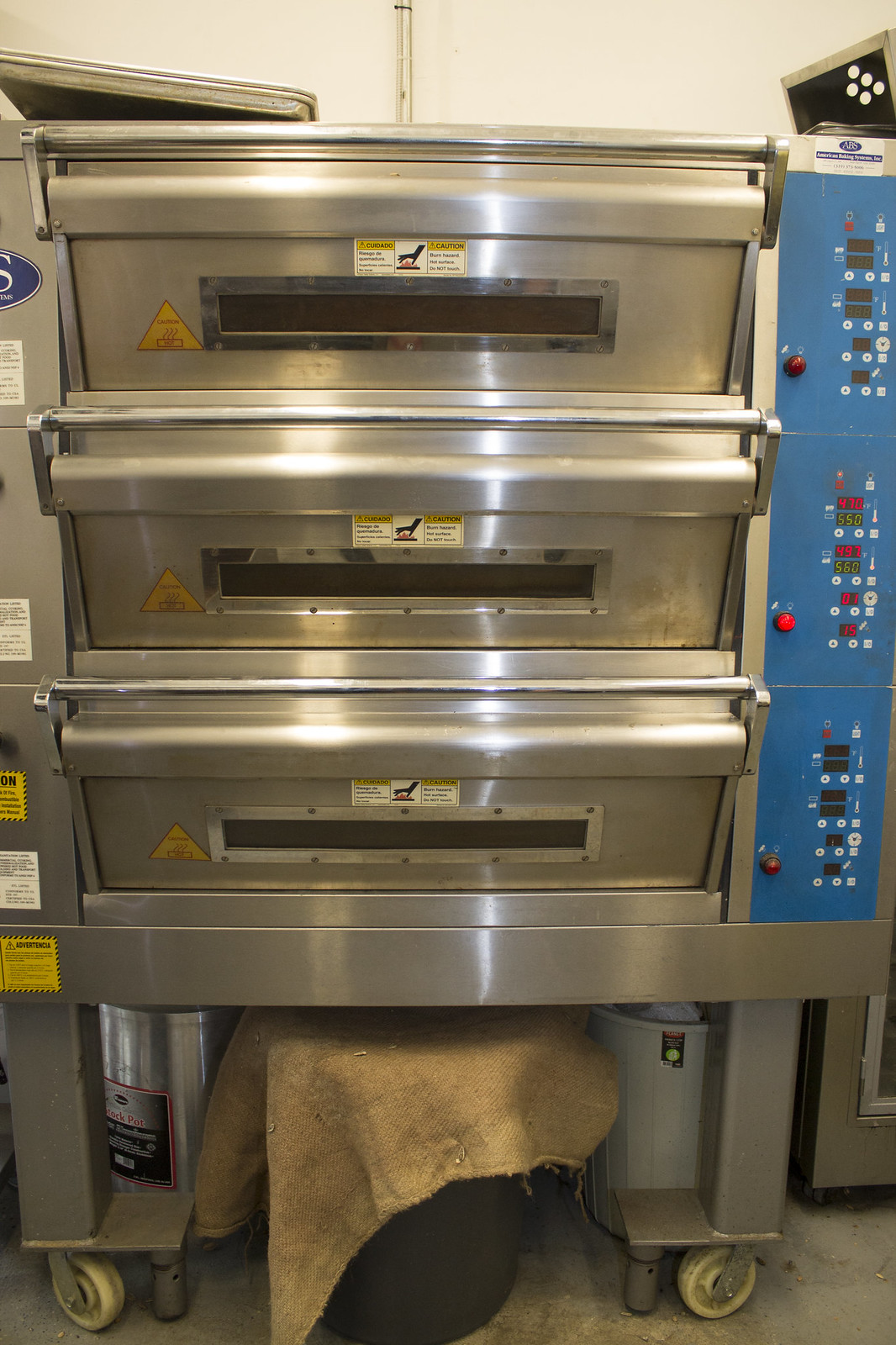This image showcases a commercial-style kitchen setup featuring a bank of three stainless steel ovens stacked on top of each other in a portrait aspect ratio. These compact ovens, which do not resemble traditional pizza ovens despite their similar shape, are fitted with blue control panels located on the right side, featuring various buttons for operation. Each oven is mounted on a mobile rack equipped with lockable wheels for stability and ease of movement. The front of the ovens displays cautionary stickers, emphasizing their industrial use. Atop the stacked ovens are two trays, while beneath them sits a black bucket covered with a piece of burlap fabric. Positioned next to the bucket is an industrial-type crock pot, and on the opposite side, there is a light gray bucket. The meticulous arrangement and specialized equipment hint at a professional kitchen environment.